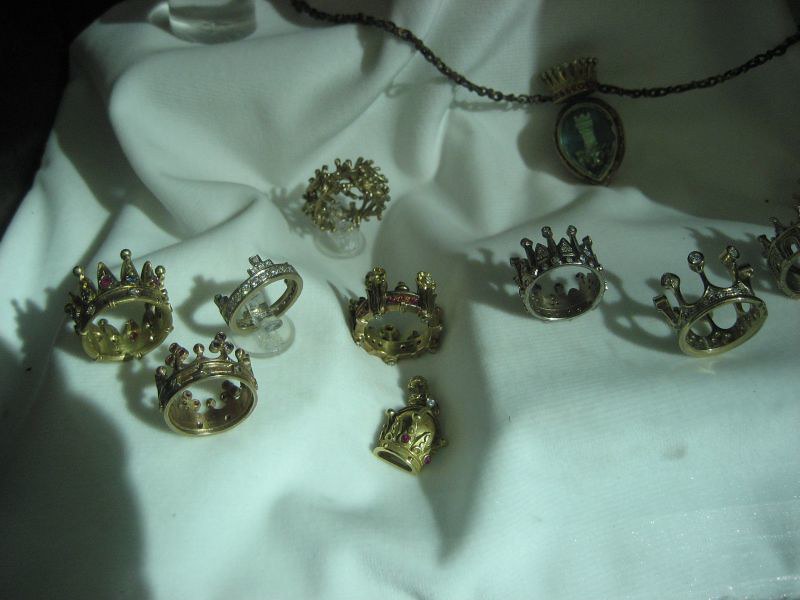This close-up photograph showcases a collection of antique, crown-shaped rings, meticulously arranged on a piece of white, silky fabric, which is possibly a drop cloth in a display case. The rings, numbering around eight to ten, vary in design and material, exuding a regal essence with their intricate details. The crowns feature a variety of royal motifs such as triangles, crosses, and tree branches, all synonymous with traditional crown shapes. The first ring is silver with sparkling crystal inlays, while the others predominantly exhibit gold hues adorned with an assortment of colored stones – including red, green, and white gems – and inlaid diamonds. Some rings resemble royal crowns with crest designs, others mimic small house roofs with steeples, and one notably looks like a small helmet accented with red gems. 

Amidst the rings, there's a notable pendant that draws attention with its unique structure – an inverted teardrop or egg shape with a tower inside, set against a blue background. This pendant is topped with a crown and is threaded through with a tarnished chain, possibly brass or black, contributing to its vintage appearance. The entire ensemble is enveloped in a shadow, possibly cast by a piece of green safety glass above the display, which gives the scene a faint bluish tint. This delicate interplay of light and shadow alongside the aged and possibly tarnished surface of the rings suggests these items have storied pasts, adding to their mystique and allure.